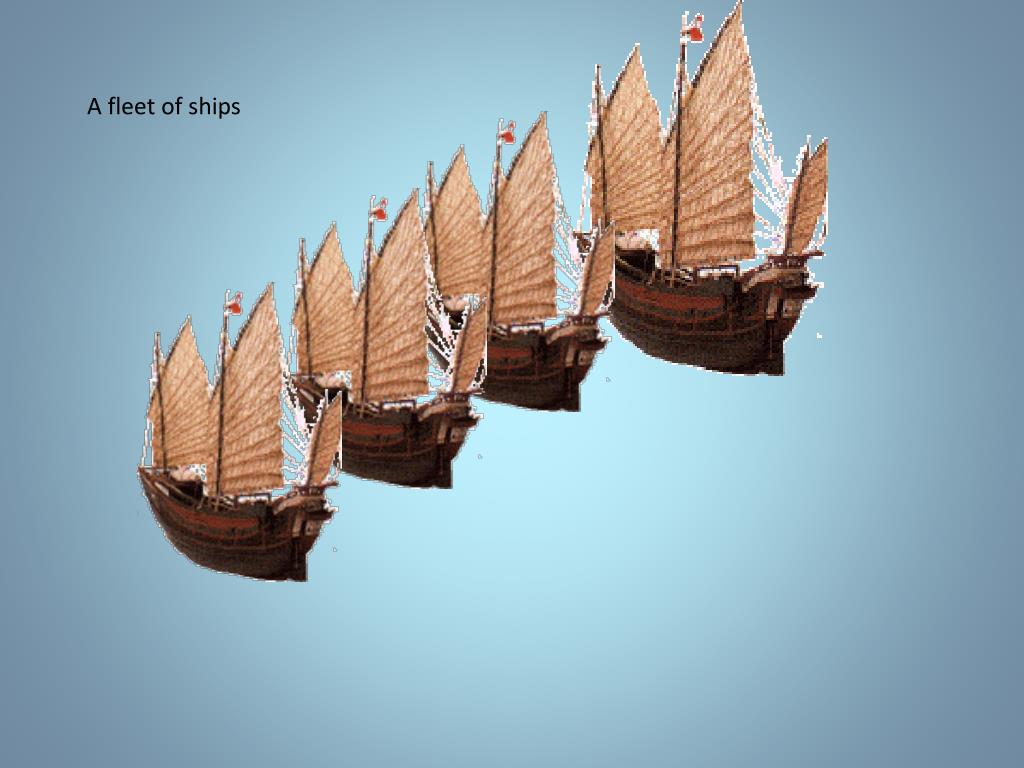The image features a pale blue background with a gradient, brightening towards the center. In the top left corner, the small black text reads "a fleet of ships." Diagonally from the bottom left to the upper right, there are four ships, each identical in design but varying in size, with the smallest placed in the lower left and the largest in the upper right. These ships have brown bodies and light tan sails, including two large sails and a tiny front sail. The middle sail of each ship has a small red and white flag. Despite the staggered appearance, the ships seem to have been crudely photoshopped onto the background, visible by the white spots around them.